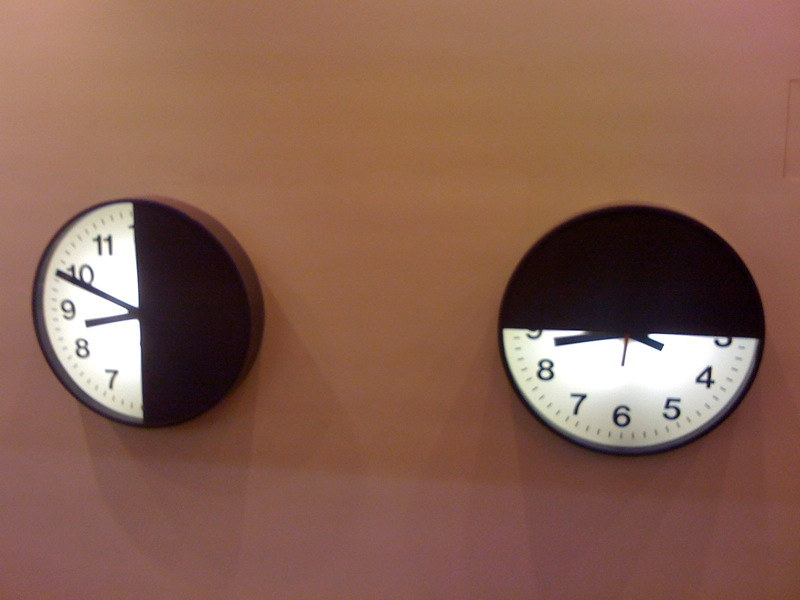This photograph captures two intriguing round clocks mounted on a dusty rose-colored wall. The clock on the left features a distinct design with a black casing and an illuminated white face. The right side of this clock's face is entirely black, devoid of any markings, while the left side maintains a traditional clock appearance with black hands, black numbers, and minute ticks. The clock on the right mirrors this unique style. Its upper half, extending from nine o'clock clockwise to three o'clock, is completely black without any indicators. The lower half is illuminated and showcases a classic white face with black hour and minute hands, black numbers, and minute notches. Both clocks display an intriguing blend of minimalist design and functionality, creating an eye-catching visual on the pastel wall.